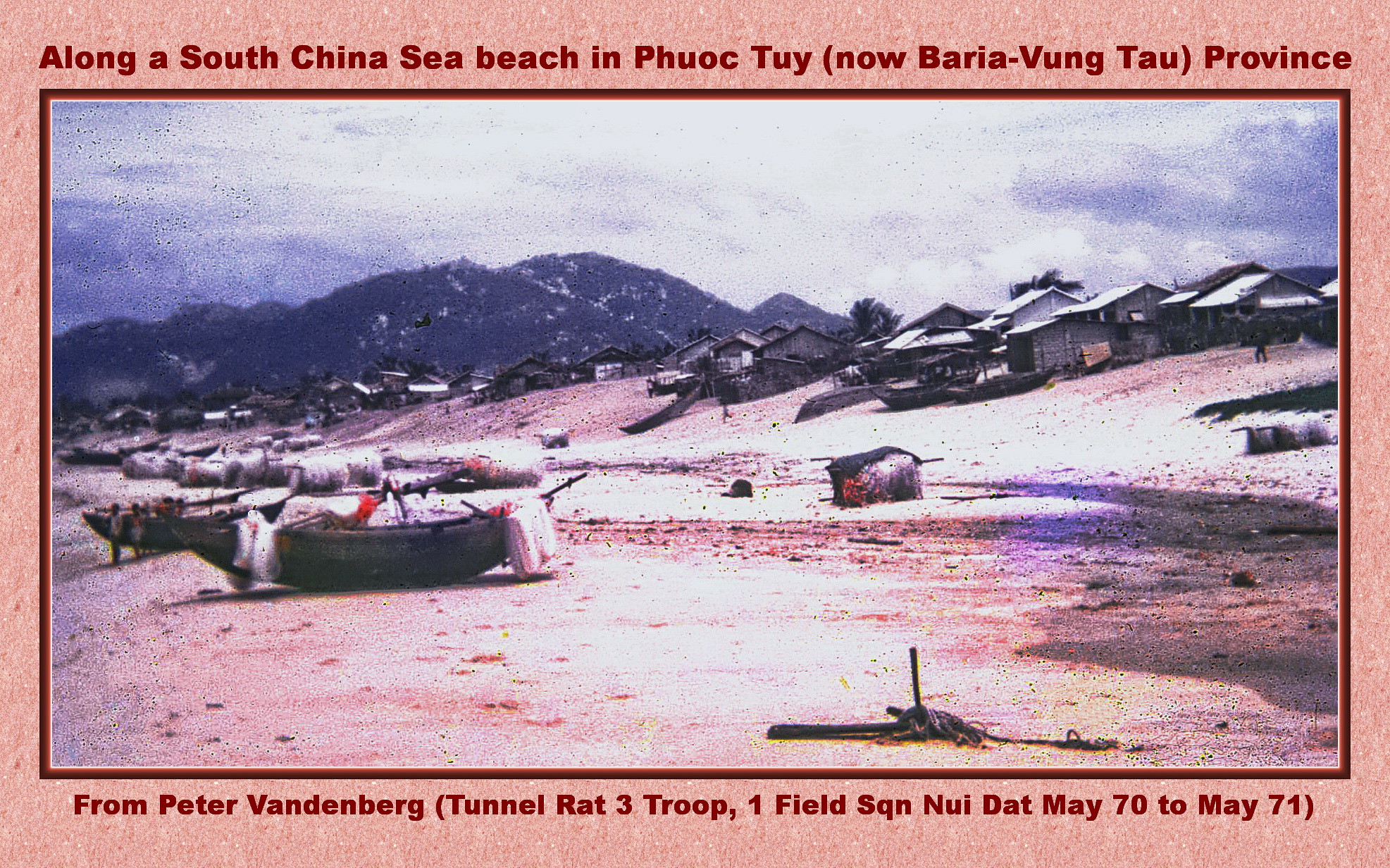This historical photograph prominently features a vast beach along the South China Sea in what is now Baria Vung Tau province, previously known as Fok Tui or Phuoc Toi. The grainy, slightly pink-tinged image, taken between May 1970 and May 1971 by Peter Vanderberg of the Tunnel Rat 3 Troop, 1 Field Squadron, captures a scene of scattered structures and objects suggesting a living or camping area. In the foreground, several wooden boats lay pulled up on the wet, sandy shore, their contents indiscernible due to the image's age and resolution. The beach, colored in earthy shades of brown and white, occupies most of the frame, and is dotted with rocks or shells. In the upper right, modest shacks sit on a hillside, while mountains with light vegetation loom in the distant background beneath a clear, blue sky. The entire scene, bordered in pink, evokes a poignant sense of history through its faded, time-worn appearance.